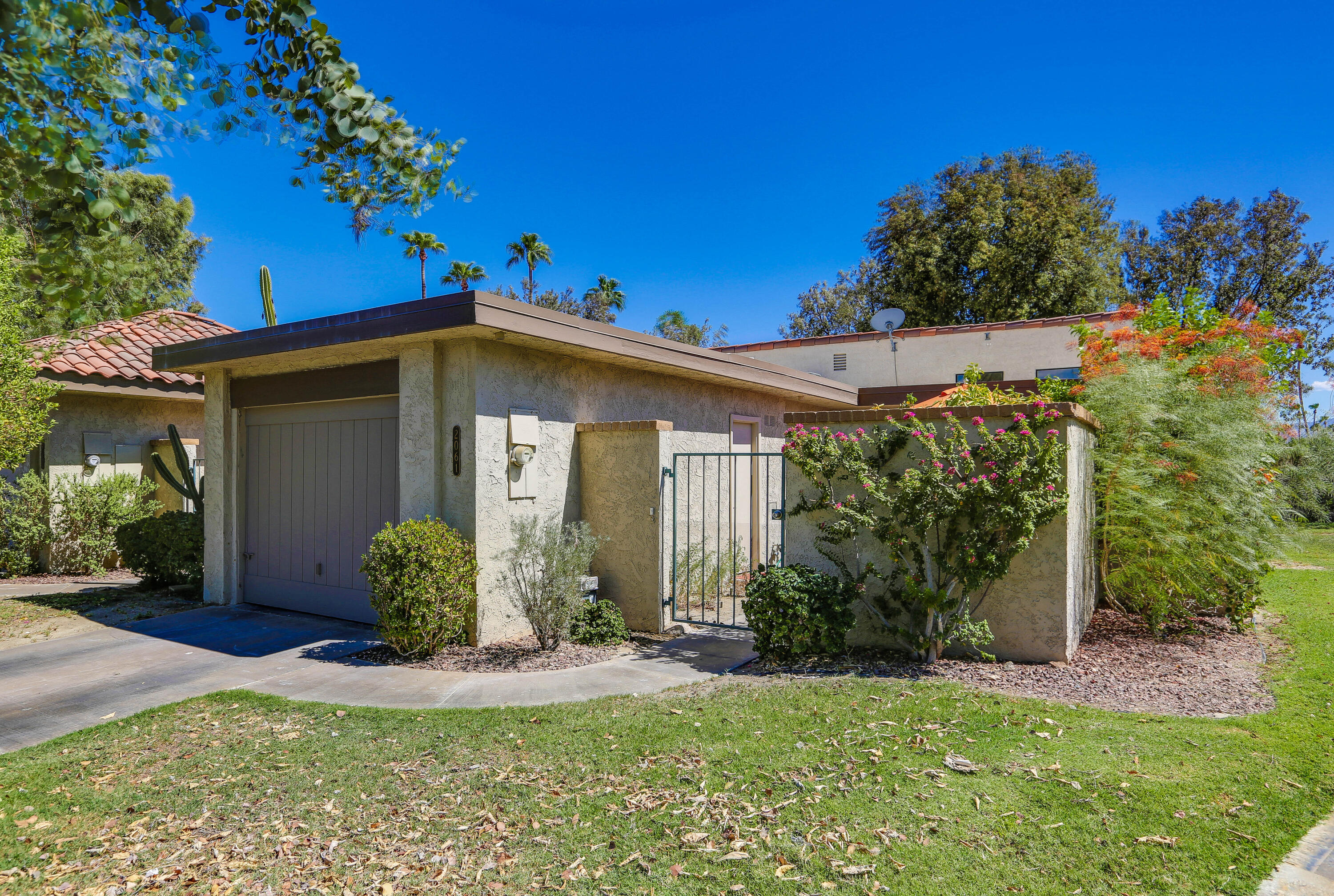This is a color photograph of a one-story home on a bright, sunny day, under a clear, deep blue sky. The house, situated in a scene reminiscent of a southwestern setting, possibly Arizona or California, features a low-ceiling and a cubic structure. A garage with a closed door is located on the left side, leading up from a driveway. To the right of the house stands a black metal gate, with a tan stone wall partially obscuring the view of the home. The front yard is well-maintained, with a neatly trimmed green lawn scattered with fallen brown leaves. Bushes with little red flowers enhance the landscape around the front of the house. Surrounding the house are several trees, their dense green foliage visible in the distance, and a particular tree to the left with a long branch extending over the roof. No people are present in the image, and the overall impression is of a quiet, sunny day with a charming, southwestern home set against a vivid blue sky.